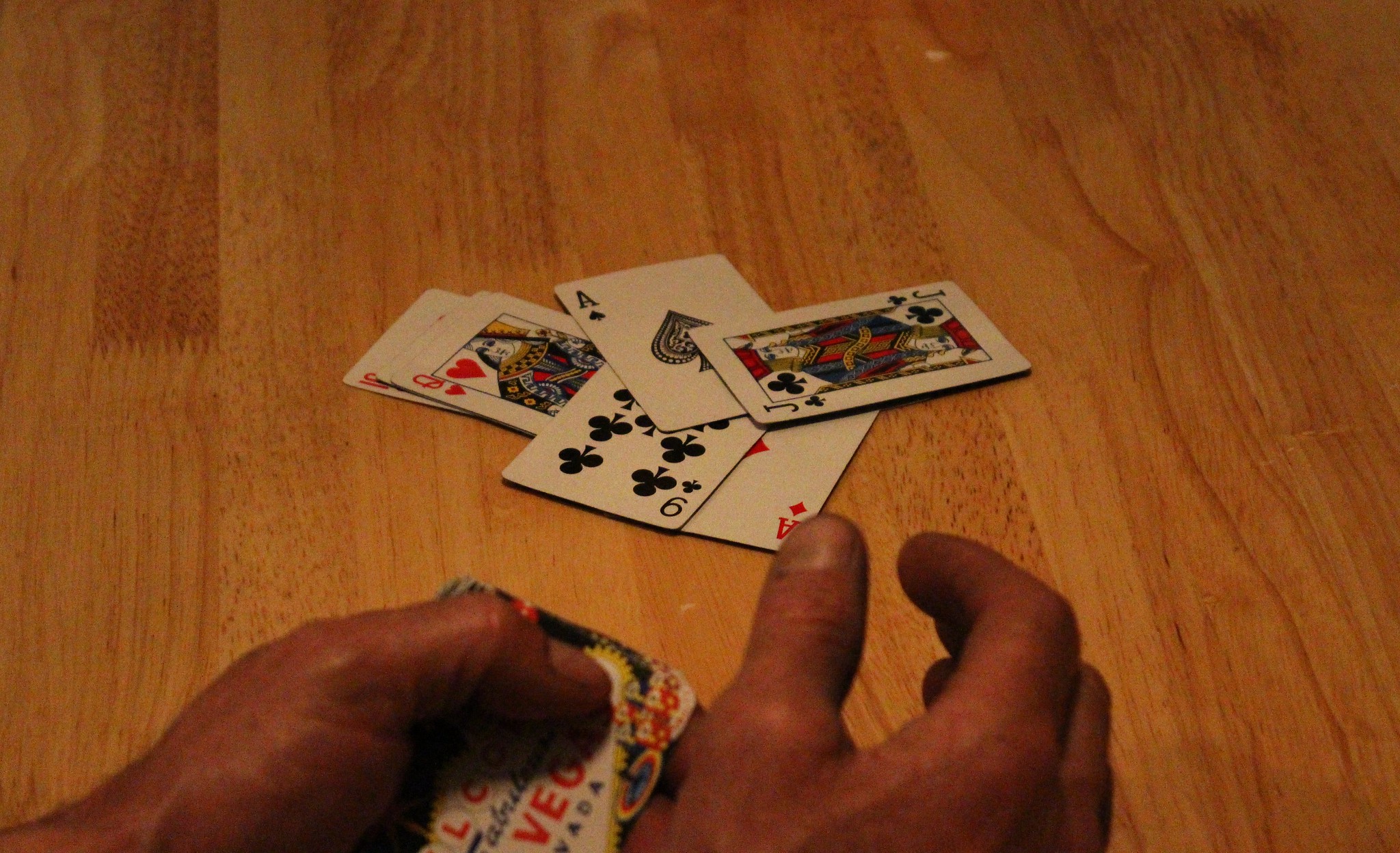In a dimly lit room, a photo captures a detailed scene at a wooden table, featuring two-toned wood with a reddish tint and a smooth, well-maintained grain. At the table sits a person, presumed to be a man based on his hands, who appears to be of African descent. His left hand holds an object that seems to be a metal tin or a playing card adorned with partial letters, "L-O" and "V-E," suggesting a Las Vegas theme.

Spread across the table are several playing cards: a Queen of Hearts, an Ace of Spades, a Nine (or possibly a Six) of Clubs, a Jack of Clubs, and an Ace of Diamonds, alongside some partially covered cards. The room's subdued lighting and the table's rich texture create a captivating contrast, emphasizing the scene's intricate details and inviting viewers to ponder the narrative unfolding in this intimate setting.